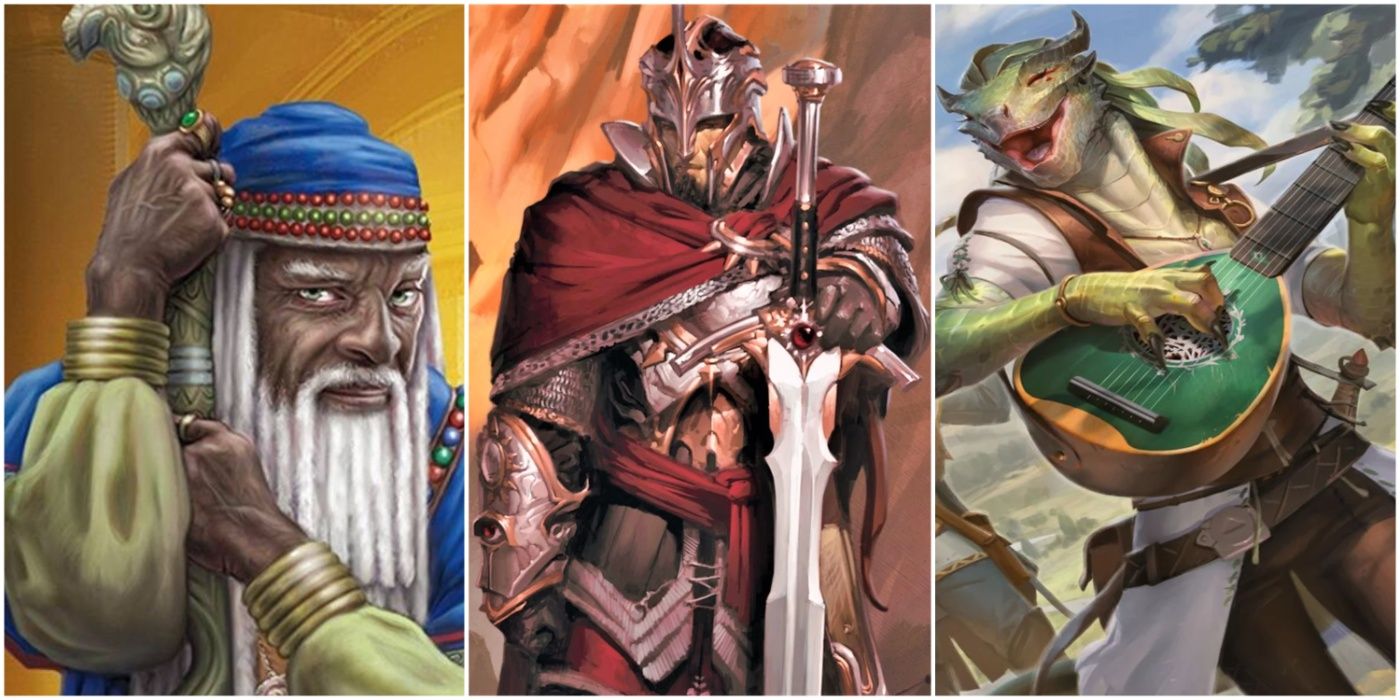The image features three vividly colored comic book or game characters, each in their own distinct setting. On the left, there's a reptilian, green monster playing a lute or mandolin, positioned outdoors. In the center, an armored knight holding a heavy sword is shown indoors or in a cave, looking off to the right. On the right, an elderly black man, possibly a genie or jester, is depicted in a close-up portrait, staring straight ahead. He wears a blue hat, has a gray beard and mustache, and holds a staff or cane. Vibrant hues of blues, reds, oranges, golds, browns, whites, and blacks are used throughout. Each character is richly detailed, with the old man adorned with rings, one bearing an emerald.